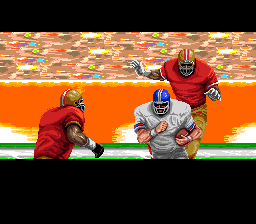The image appears to be an artistic rendering from a video game, depicting an intense football scene. The background showcases an orange wall with gold trim, positioned in front of a grandstand bustling with spectators, illustrated as a mix of brown with tiny vibrant specks of blue, green, white, and red. On the left side, a football player in a red jersey stands prominently, donning a gold helmet with a red stripe. His muscular arms are visible and covered in white and black gloves. Toward the center, another player in a gray jersey with red and blue arm stripes is seen from the front, wearing a blue helmet featuring a red and white stripe and a face guard. He clutches a brown football in his left arm. Another player, similarly attired in a red jersey and gold helmet with a red stripe, and gold pants, appears to be in pursuit of the one carrying the football. The scene is framed with a black border at the bottom.